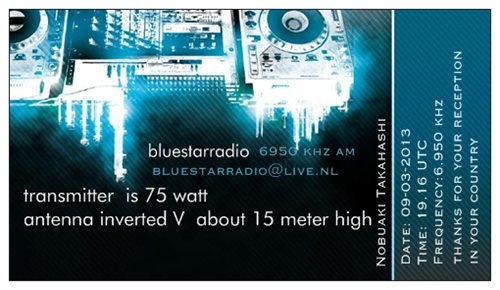This image resembles a flyer or business card with its rectangular format, featuring a dark blue, black, teal, and white color scheme. At the top, there are visuals of a DJ mixing station with two turntables flanking a central mixing board, enhanced by a half-tone scanline filter. The main text is prominently displayed in white and reads: "Blue Star Radio, 6950 KHz AM, bluestarradioatlive.nl." 

Below this, additional details are provided: "Transmitter is 75 watts, antenna inverted V about 15 meters high." Along the right side of the image, oriented vertically, it reads: "Nobuaki Takahashi, date 09/03/2013, time 1916 UTC, frequency 6950 KHz." The caption concludes with, "Thanks for your reception in your country." 

Overall, the composition conveys an advertisement or confirmation of a radio transmission, characterized by both technical specifications and a personal touch.